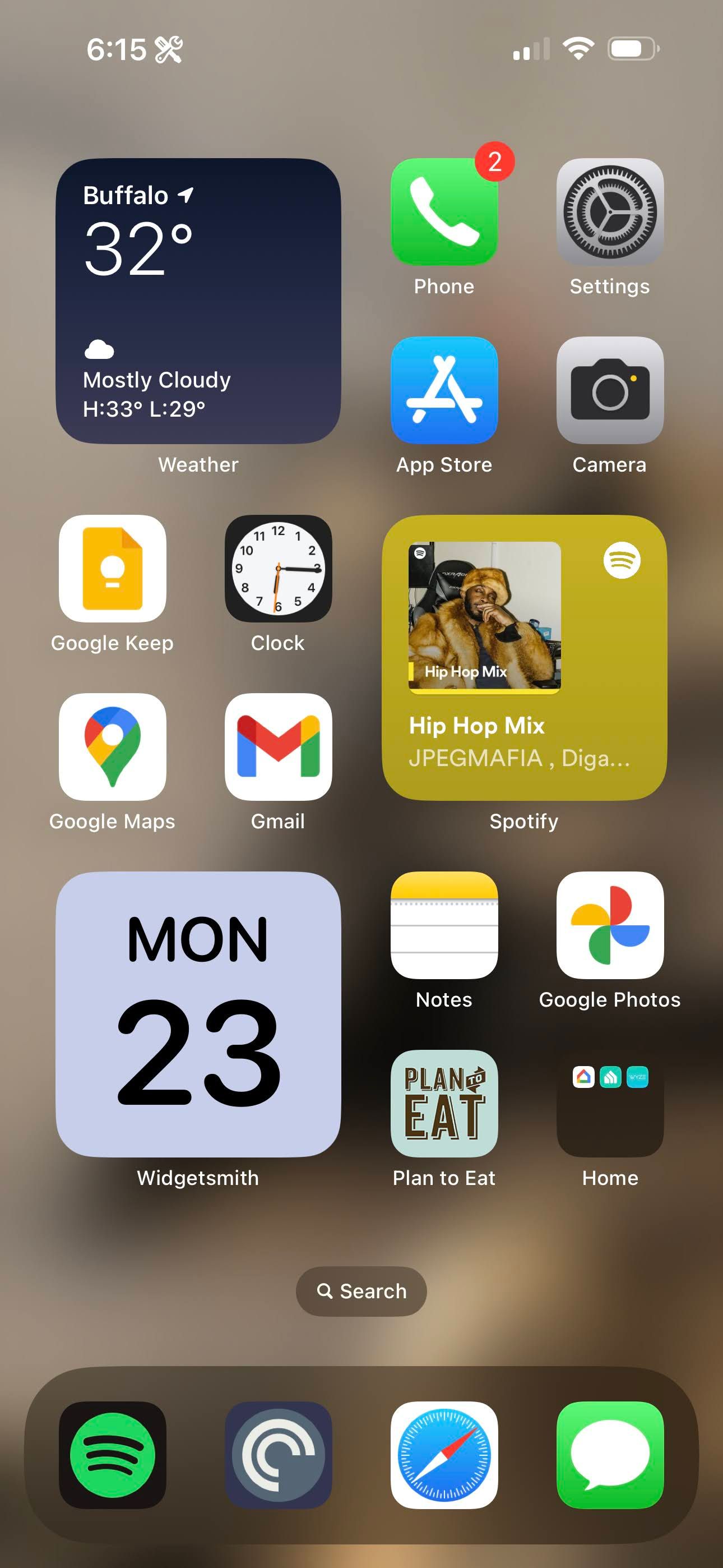The screenshot is of an iPhone home screen with the time displayed at the top left corner as 6:15. Just to the right of the time, there is an icon of a crossed screwdriver and wrench, forming an X, indicating some sort of system or settings app. Proceeding further to the right, the status bar shows two out of four cellular signal bars, a full three-bar Wi-Fi signal, and a battery meter that appears to be about 82% full. The background is a blurred light brown or bronze color.

The weather widget indicates the location is Buffalo, with the active locator icon (an upwards pointing arrow) next to the name. The temperature is shown as 32°C with a mostly cloudy forecast, a high of 33°C, and a low of 29°C.

On the home screen, the Phone app displays two notifications. Following this, the Settings app is visible, followed by the App Store icon below it. The Camera app is also on this screen. The Spotify app shows the currently playing album "HipHopMix" by JPEGMAFIA. 

To the left side of the screen, there are apps for Google Keep, Clock, Google Maps, and Gmail. The date displayed on the Widgetsmith app reads Monday the 23rd. To the right of Widgetsmith, there are apps for Notes, Google Photos, Plan to Eat, and Home.